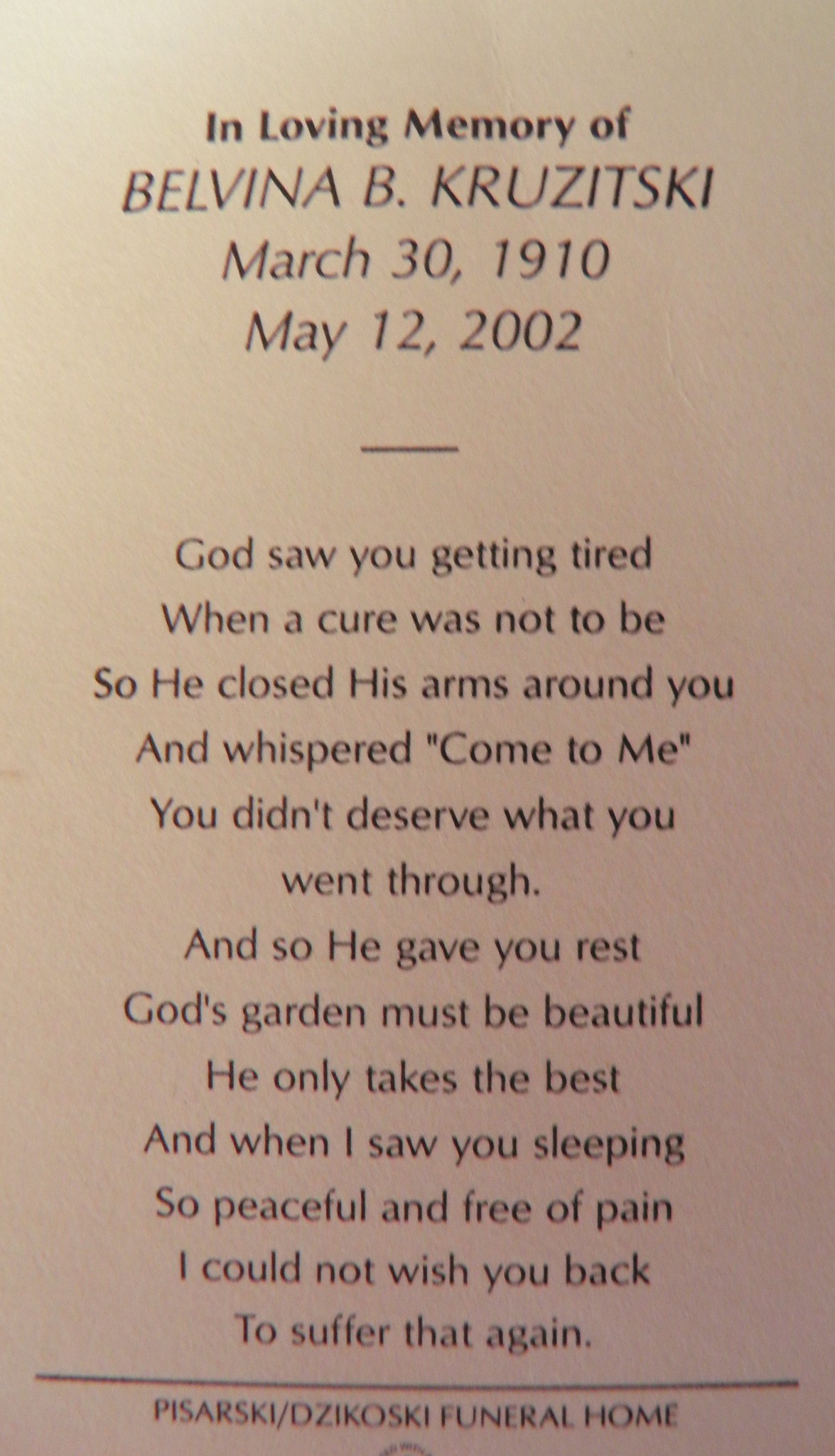This image is a vertical, rectangular tribute featuring an obituary or poem in honor of a recently deceased individual. At the top, it reads, "In loving memory of," followed by the name "Balvina B. Krasitsky" (March 30, 1910 - May 12, 2002) in larger letters. Beneath the dates is a heartfelt poem: 

"God saw you getting tired when a cure was not to be, so He closed His arms around you and whispered, 'Come to me.' You didn't deserve what you went through, so He gave you rest. God's garden must be beautiful. He only takes the best. And when I saw you sleeping so peaceful and free of pain, I could not wish you back to suffer that again."

The text is centered against an elegant background, with an off-white or pink hue, perhaps symbolizing serenity. The image contains no other objects, maintaining a solemn and respectful tone. At the bottom, the name of the funeral home that printed this memorial is listed. This entire presentation serves as a dignified tribute to the memory of Balvina B. Krasitsky.